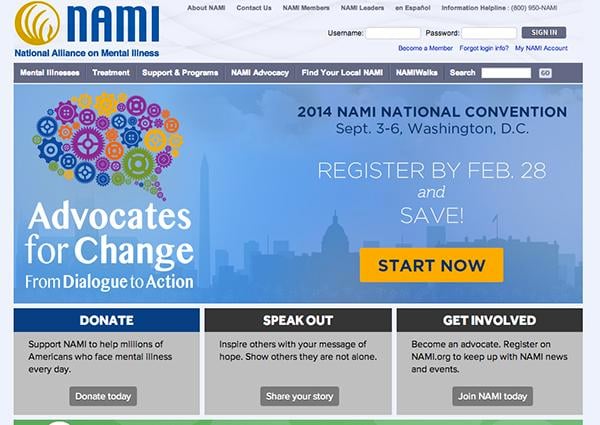This is a screenshot of the NAMI (National Alliance on Mental Illness) website. The header is in light gray and features intricate, curvy, criss-cross patterns. The website name "NAMI" is prominently displayed in blue text, accompanied by a gold logo resembling a stylized hand. Below the name, the organization's full title, "National Alliance on Mental Illness," is written in smaller blue text.

Just beneath the header, there is a dark gray menu strip with white text. The menu options include "Mental Illness," "Treatment Support and Programs," "NAMI Advocacy," "Find Your Local NAMI," and an option that appears truncated as "NAMI Walls." At the end of this strip, there is a search box.

The main content of the page features a blue background with a darker blue silhouette of the Washington, D.C. cityscape. In white text, it declares "Advocates for Change," and above this text, there is an artistic brain shape formed by colorful, interlocking gears. The page prompts users to "register by February 28th and save, start now."

Below this central section, there are four gray panels, each with black or blue headers, providing options to donate, speak out, and get involved. For additional information, visitors are directed to the website www.NAMI.org.